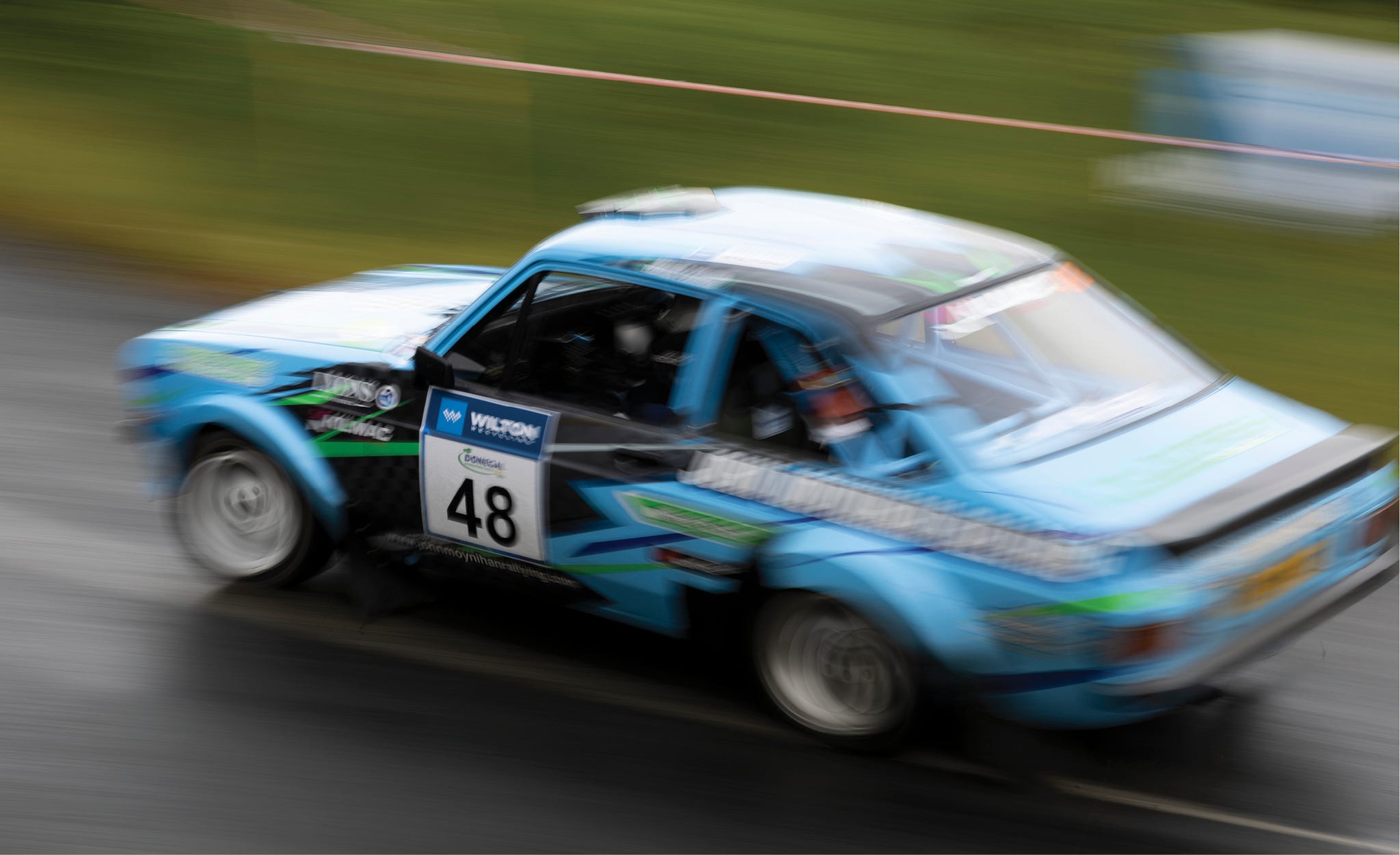In this image, we see a blurry, older-style rally race car from the 1970s or 1980s speeding on a track. The car, primarily blue with black accents along the door and some green streaks, has the name "Wilton" and the number "48" prominently displayed on a white placard affixed to its side. The driver is partially visible inside. The car is surrounded by various, undecipherable advertisements due to the motion blur. The road it races on appears to be asphalt with a dividing white line, and is accompanied by a backdrop of green grass, albeit blurred. A beige streak runs across the upper part of the image from right to left, adding another layer to the dynamic scene.